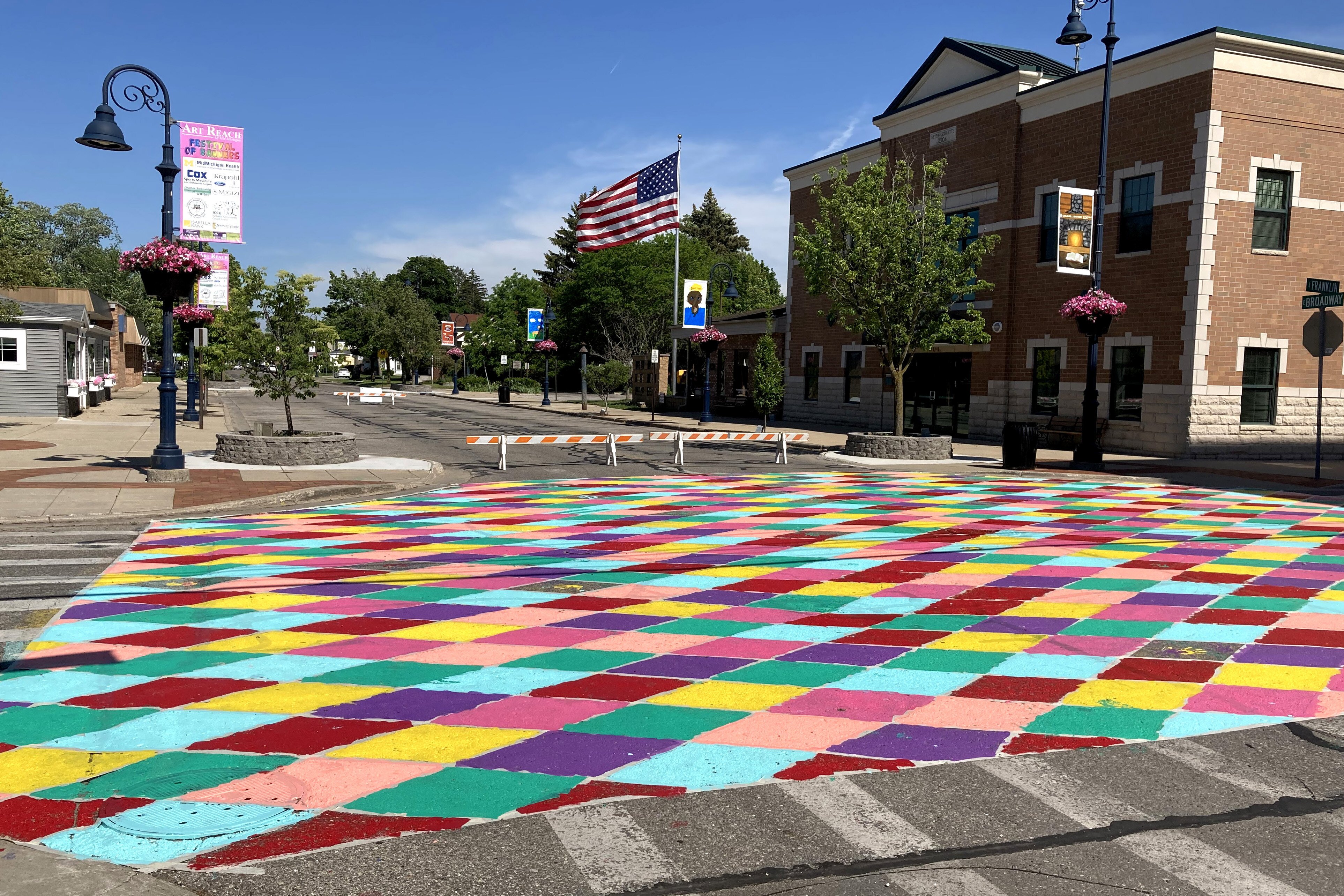The photograph depicts a brightly lit intersection in a small town, observed on a clear day under a blue sky dotted with white clouds. The focal point of the image is a road colorfully painted with interconnecting diamond-shaped patterns in a vibrant array of colors including green, peach, yellow, red, purple, blue, light pink, and dark pink. The road appears to be closed off by horizontal orange and white striped barricades.

At the lower right-hand side of the image, a white crosswalk traverses the road from left to right, mirrored on the center-left side of the street. Surrounding the intersection are multiple light poles adorned with hanging flowers. 

To the right side of the road stands a prominent red brick building, two to three stories tall, which is flanked by an American flag mounted on a pole. In front of the building, the sidewalk is lined with large green trees. 

In the upper left corner, a gray sidewalk accompanies additional gray buildings, contributing to the townscape. The setting is thoroughly bathed in natural light, enhancing the vibrant colors and details of the serene small-town environment.